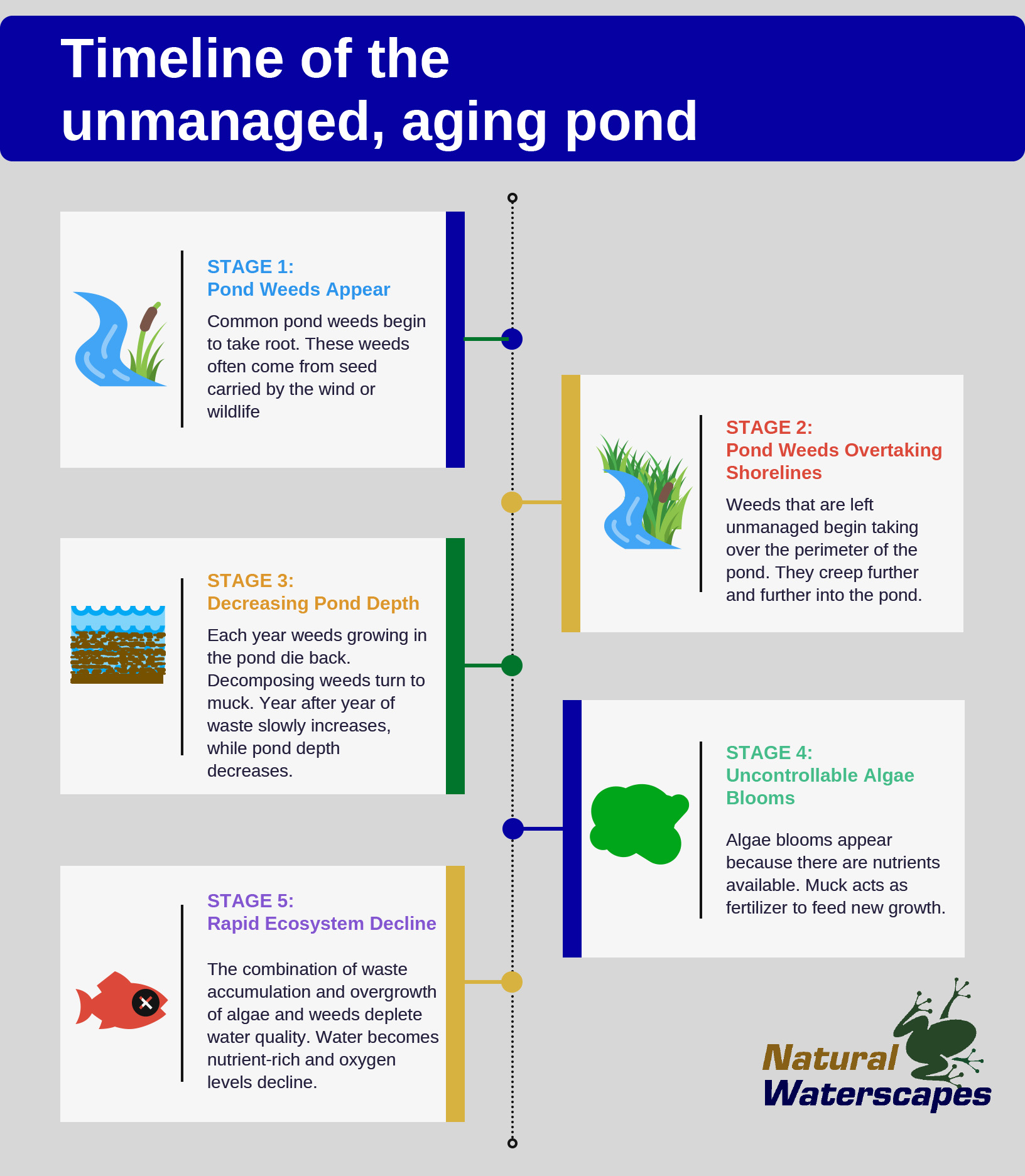The infographic by Natural Waterscapes, titled "Timeline of the Unmanaged Aging Pond," reveals a detailed progression of pond degeneration through five distinct stages. The title's words are color-coded, with "Natural" in brown, "Waterscapes" in purple, and an outline of a frog beside them. The infographic includes rich, colorful illustrations representing each stage of pond aging. 

Stage One shows the onset of pond weeds, which take root from seeds often dispersed by wind or wildlife. An image depicts a pond with characteristic green vegetation and little brown cattails. 

Stage Two illustrates the encroachment of weeds over the shorelines, gradually dominating the pond's perimeter. The associated image shows increased greenery spreading around the pond's edges. 

Stage Three details the reduction in pond depth due to the accumulation of decomposing weeds, visible in a side-view diagram highlighting muck buildup and diminishing water levels.

Stage Four focuses on uncontrollable algae blooms, spurred by nutrient-rich muck acting as fertilizer for new growth. The corresponding image is dominated by green algae bloom, almost overtaking the visual.

Stage Five describes the rapid ecosystem decline where accumulated waste and overgrowth deplete water quality and oxygen levels, depicted by a red fish with a black X over its eye symbolizing deterioration.

The entire infographic serves as an educational tool, vividly demonstrating the unchecked progression of pond aging.